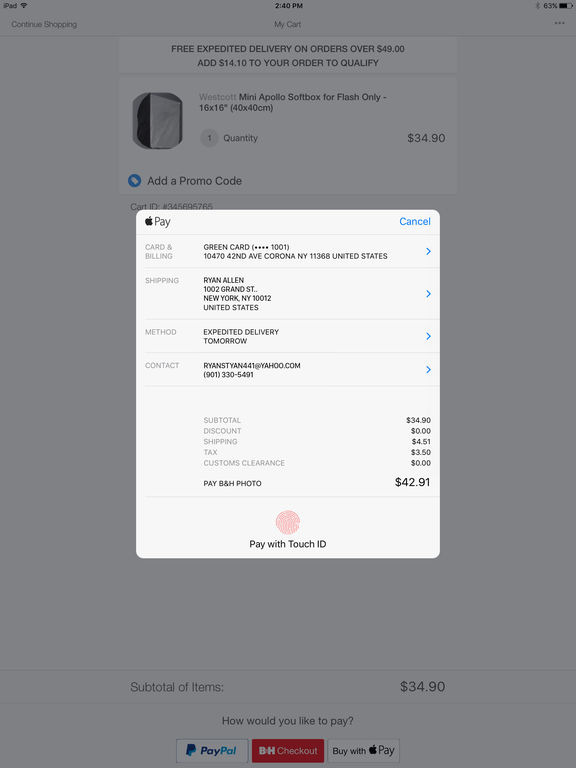A detailed invoice is displayed on a tablet. The screen indicates a Wi-Fi connection, with the current time at 2:40 PM, battery level at 63%, and Bluetooth enabled. The main section of the invoice shows a cart summary, highlighting a special offer of free expedited delivery on orders over $49. The current order, totaling $34.90, includes one item: a Westcott Mini Apollo Softbox for Flash (16x16). There is an option to add a promo code.

Below the itemized list, there is a semi-transparent overlay with a pop-up window featuring Apple Pay as a payment option on the left, and 'Cancel' on the right. The billing information reads: Green Card ending in 1001, registered to an address at 1047 2nd Avenue, Corona, New York, 11368, United States. The shipping information is listed as: Ryan Allen, 1002 Grand Street, New York, New York, 10012, United States. The shipping method selected is expedited delivery, promising arrival by tomorrow. The contact details provided are for Ryan Styan, with the email ryanstyan441@yahoo.com and phone number 901-330-5491.